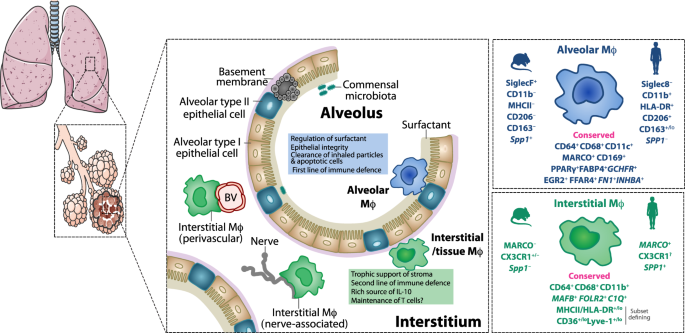The image is a detailed medical infographic focused on the lungs. On the upper left corner, there's a drawing of a pair of lungs in pink, with a small square highlighting a segment of the lung tissue. This highlighted area is further expanded into a larger box, showing a magnified view of the alveoli, the tiny air sacs in the lungs. Within this expanded section, a further zoomed-in area details the cellular structure and membranes of the lung sacs, labeled with terms like basement membrane, conventional microbiota, alveolus, alveolar surfactant, and various types of cells and membranes. Specific labels identify components such as alveolar type 1 epithelial cell, alveolar type 2 epithelial cell, nerve cells, and structures within the interstitium. Green blotch markers identify interstitial MO, with other areas labeled as alveolar MO and interstitial MO. This scientific illustration seems to be designed to showcase the intricate details of lung anatomy at a microscopic level.